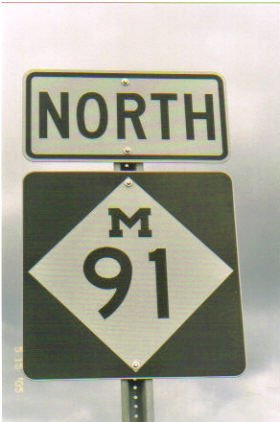The image depicts a roadside sign mounted on a steel post. The post is designed with holes along its length, suggesting a perforated bracket structure that aids fastening. At the base, two flat steel flanges extend outward, likely for securing the post to the ground with bolts or other fasteners.

The main feature of the sign is a square black background adorned with a white diamond in the center. Inside this diamond, white characters display "M91". Above this square sign, there is a horizontally long, vertically narrow, rectangular white sign with a black border. This sign reads "NORTH" in black characters, indicating directional information.

Visible silver-toned fasteners secure both signs to the post, providing a sturdy assembly. The backdrop of the scene features a very gray, overcast sky, adding a somber tone to the overall image.